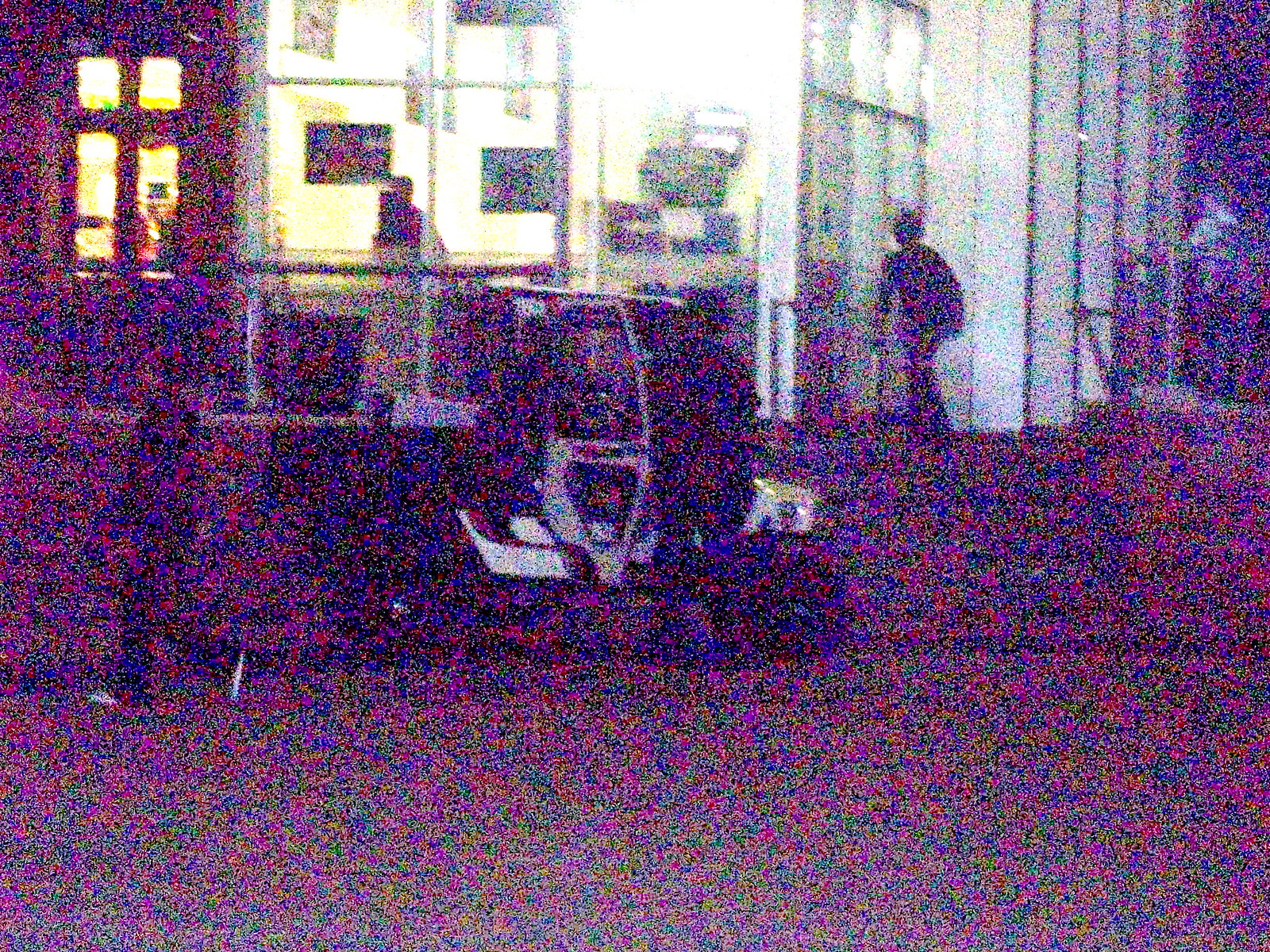The grainy, low-resolution image appears to depict an urban outdoor setting, possibly taken from security footage. At the center of the scene, there is a small, motorized golf cart-like vehicle with a white frame and large tires, positioned on a concrete road. A person is seen next to the golf cart, and another one is walking towards the left edge of the image. In the background stands a large building featuring numerous windows and steps leading up to multiple doorways. One person is visible walking up the steps to the right, while another is near a doorway on the left emitting a yellow light. The far-right section of the image shows an individual against a dark background. The image's poor quality makes further details hard to distinguish.